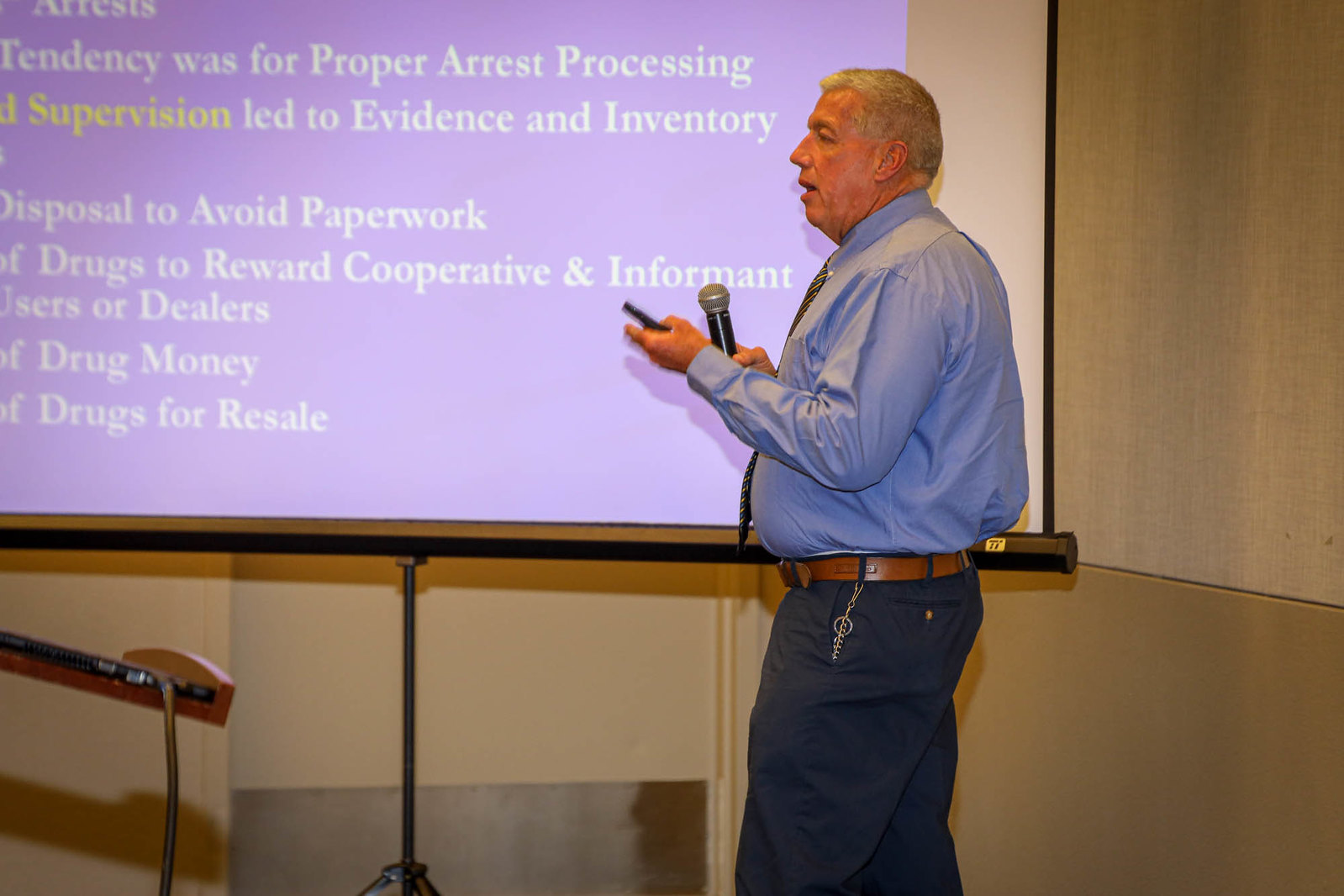The photograph captures a man delivering a solo presentation in what appears to be either a conference room or classroom with tan walls. He stands poised with a serious expression, looking slightly to his left at a projector screen, which displays a slide with blue background and white lettering, highlighted with yellow. Key visible words on the slide include "drugs," "supervision," "evidence," "inventory," and phrases like "to avoid paperwork," and "drugs for resale," indicating a topic related to drug enforcement or police procedures. The man is dressed in a blue button-down shirt, dark blue pants, a tie, and a brown belt, holding a microphone in one hand and a remote control for the slides in the other. The setting and content suggest he might be instructing an audience, possibly law enforcement officers, on proper arrest processing and evidence management.